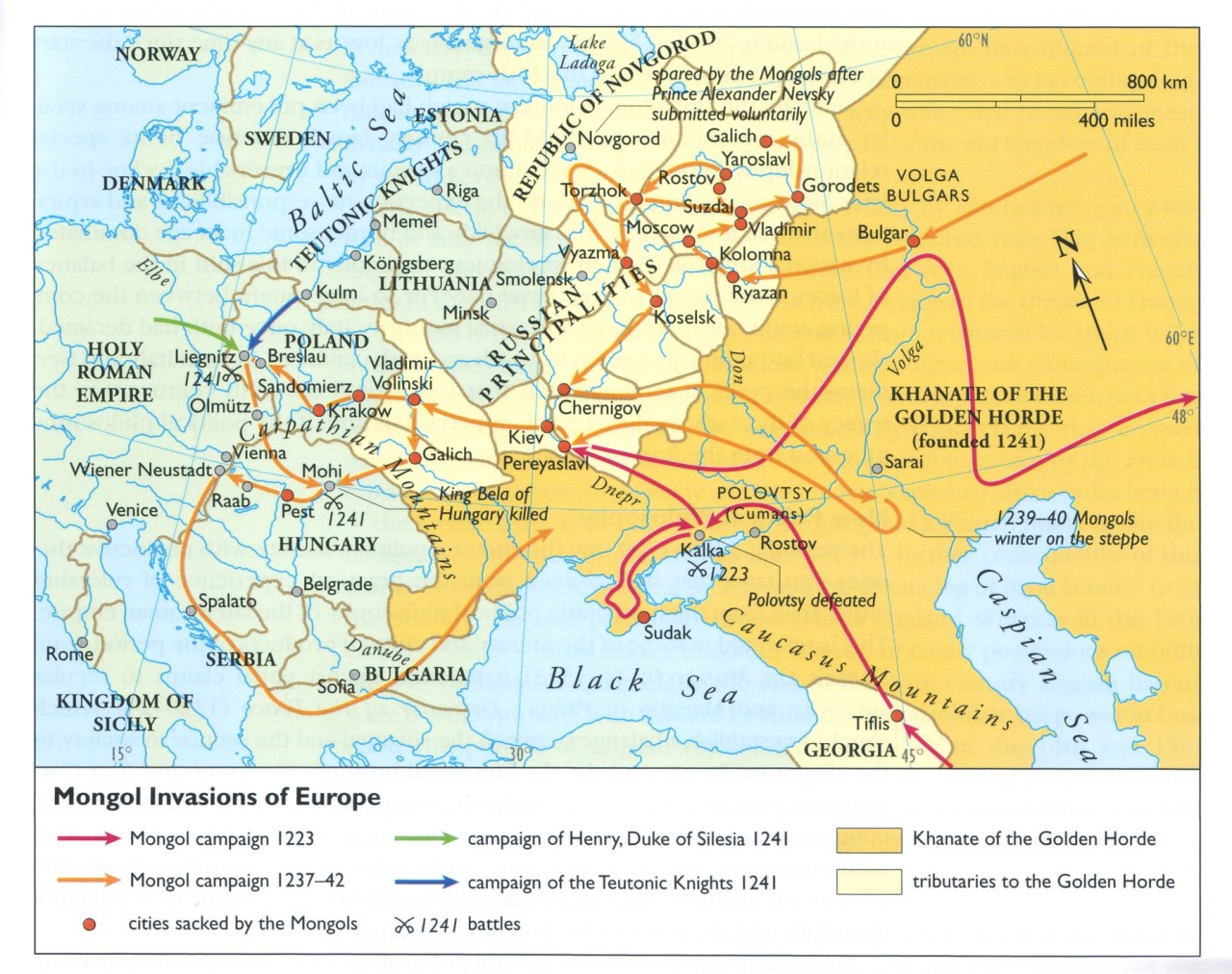This is a detailed color map illustrating the Mongol invasions of Europe. The map prominently features regions including Georgia, Bulgaria, the Russian Principalities, Estonia, Hungary, Serbia, the Holy Roman Empire, and the Kingdom of Sicily. Various other regions, such as Norway, Sweden, Denmark, the Republic of Novgorod, and Siberia, are also marked.

Overlaid on the map are colored arrows and symbols detailing the Mongol campaigns. Red arrows indicate the Mongol Campaign of 1223, while orange arrows specify the Mongol Campaign from 1237 to 1242. Green arrows denote the Campaign of Henry, Duke of Silesia, in 1241, and blue arrows highlight the Campaign of the Teutonic Knights in 1241. Red dots mark the cities sacked by the Mongols, and cross swords symbolize battles in 1241.

The map also uses color shading to illustrate territorial control: deep golden indicates the Khanate of the Golden Horde, founded in 1241, and light yellow shows tributaries to the Golden Horde. The Black Sea is visible in blue, providing a notable geographic reference point.

At the bottom of the map is a wide white stripe containing the key, which is rendered in black text and provides explanations for the various arrows and markers used throughout the map. The landmasses are depicted in different shades of tan, making the colored lines and symbols stand out against the background.